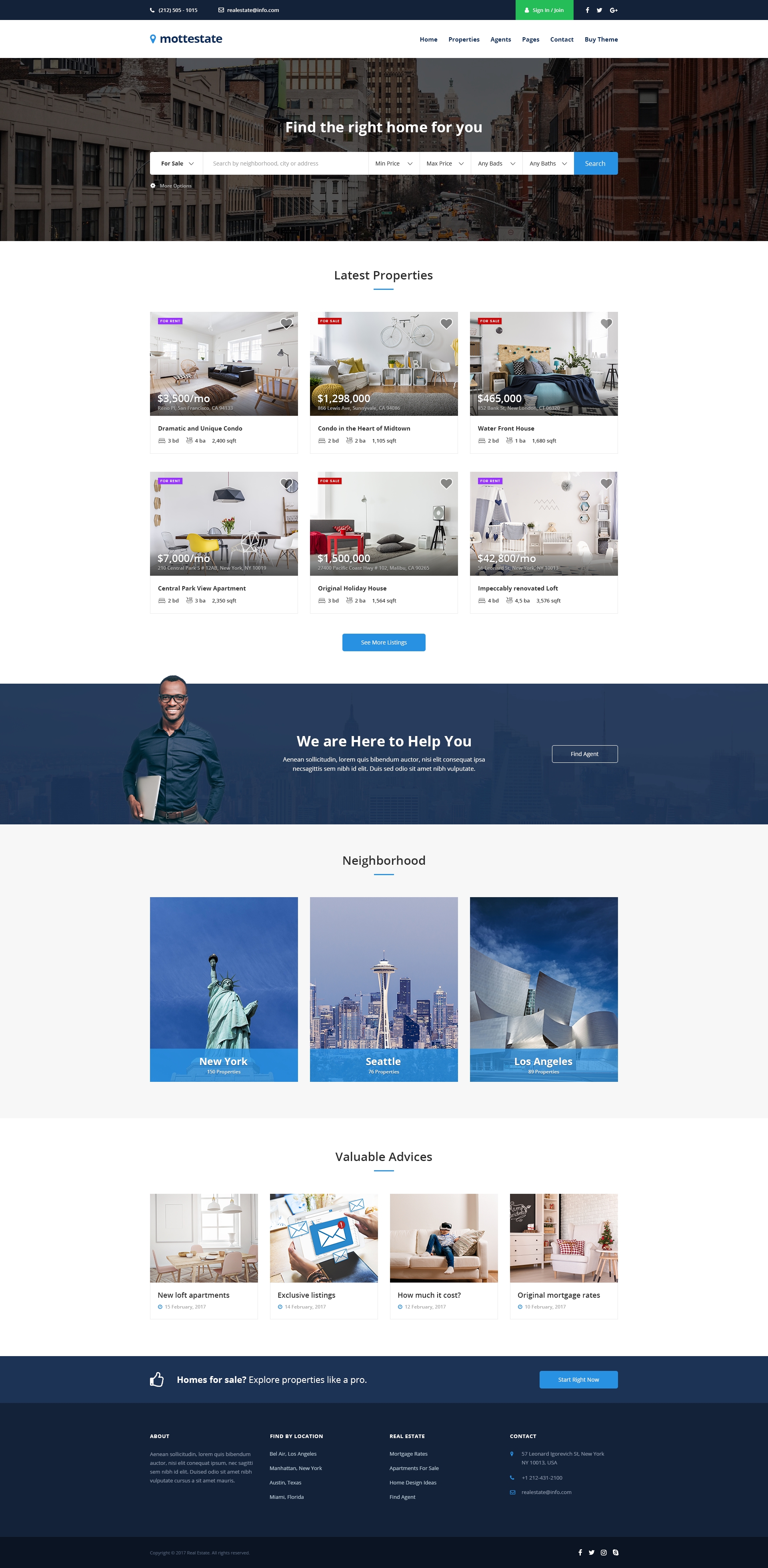The image depicts a sleek, modern website interface for 'Mottestate'—a real estate theme designed for home finding. In the upper left corner, the branding 'Mottestate' (M-O-T-T-E-S-T-A-T-E) is prominently displayed. The top of the site features a black navigation strip. On the left side of this strip are numbers '2-1-2-5-0-5-10-15' and an email address 'realestateatinfo.com'. 

On the right side, there are options to 'Sign In' or 'Join', and a green button with white text. Adjacent to these are icons for social media platforms Facebook, Twitter, and Google+.

Below this top strip, a wider white strip displays the 'Mottestate' brand again, with main navigation options to the right: 'Home', 'Properties', 'Agents', 'Pages', 'Contact', and 'Buy Themes'. This clues us in that the site is designed as a theme, rather than an actual real estate marketplace.

The main header image is a grayscale photograph featuring a downtown area with tall buildings lining a street. Overlaying this image is large white text that reads 'Find the right home for you.' Below this header, there is an intuitive search bar allowing users to search for properties. The search options include dropdown menus for 'For Sale', search by 'Neighborhood, City, or Address', 'Minimum Price', 'Maximum Price', 'Any Beds', and 'Any Baths'. To finalize the search, a conspicuous blue search button is located at the end of the bar.